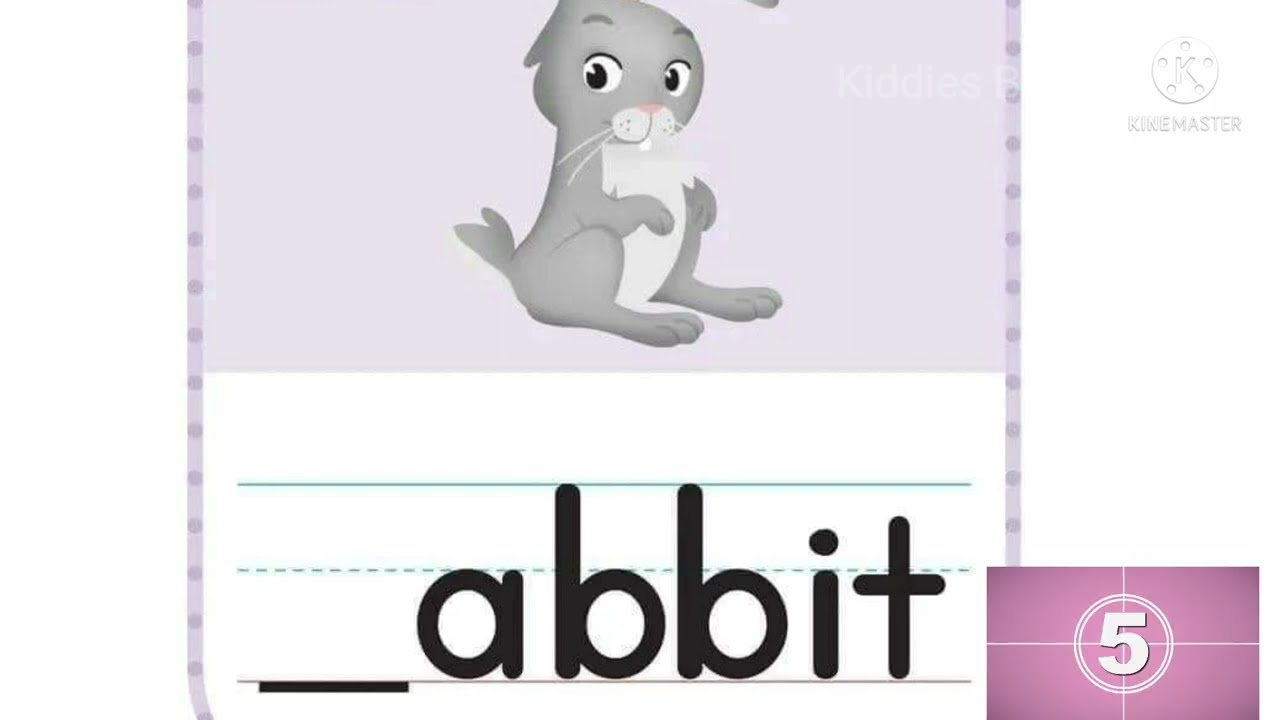This image depicts an educational card for teaching children how to spell words, specifically the word "rabbit." At the top, the text "Kitties Bee" is displayed with a pale and blended background, followed by "K-I-K-E Master" with the letter "K" circled and accompanied by five white dots. The main illustration is a cartoon gray rabbit with a white belly, sitting with its body facing to the right and its large googly eyes looking directly at us. The rabbit has a small pink nose, long white whiskers, a single visible white tooth, and a fluffy lining under its head.

Below the rabbit, there's a section resembling notebook paper with green top and dotted lines, and another straight green line below them, creating a place for children to practice writing. The word "A-B-B-I-T" is written on this lined area, with a blank space before the "A" to prompt children to fill in the missing letter "R."

To the bottom right of this writing section, there's a small pink rectangle with the number "5" in the center, circled and possibly signifying a countdown timer. The overall background is gray, adding a subtle contrast to the elements of the educational card.